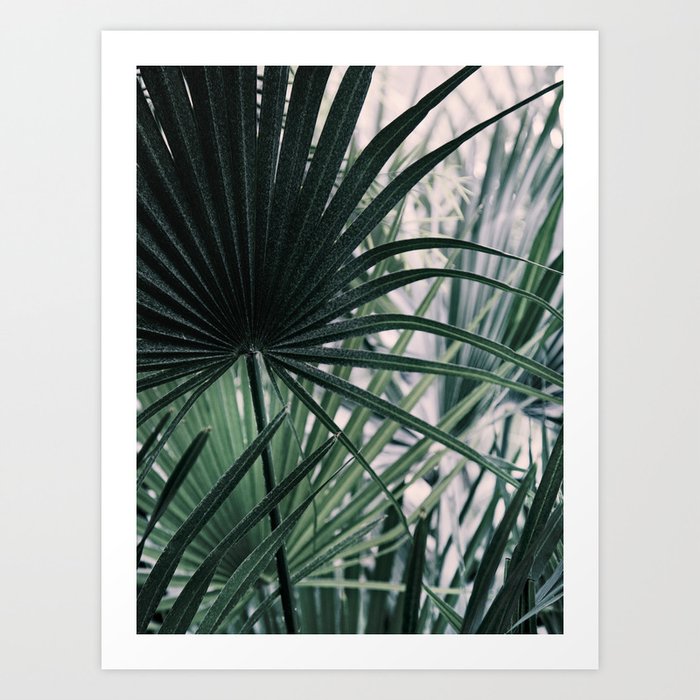The image displays an art print on a light grey wall, featuring vibrant green plants with long, thin stems and fan-like clusters of leaves, reminiscent of tropical or palm species. The print is surrounded by a white border and framed with a grey rectangle, maintaining a clean aesthetic. The background of the print includes lush greenery and a white sky, enhancing the vividness of the dark and light green leaves. The arrangement of the plants shows varying sizes and hues, creating a visually appealing, multi-layered composition that evokes the serenity of a green room.